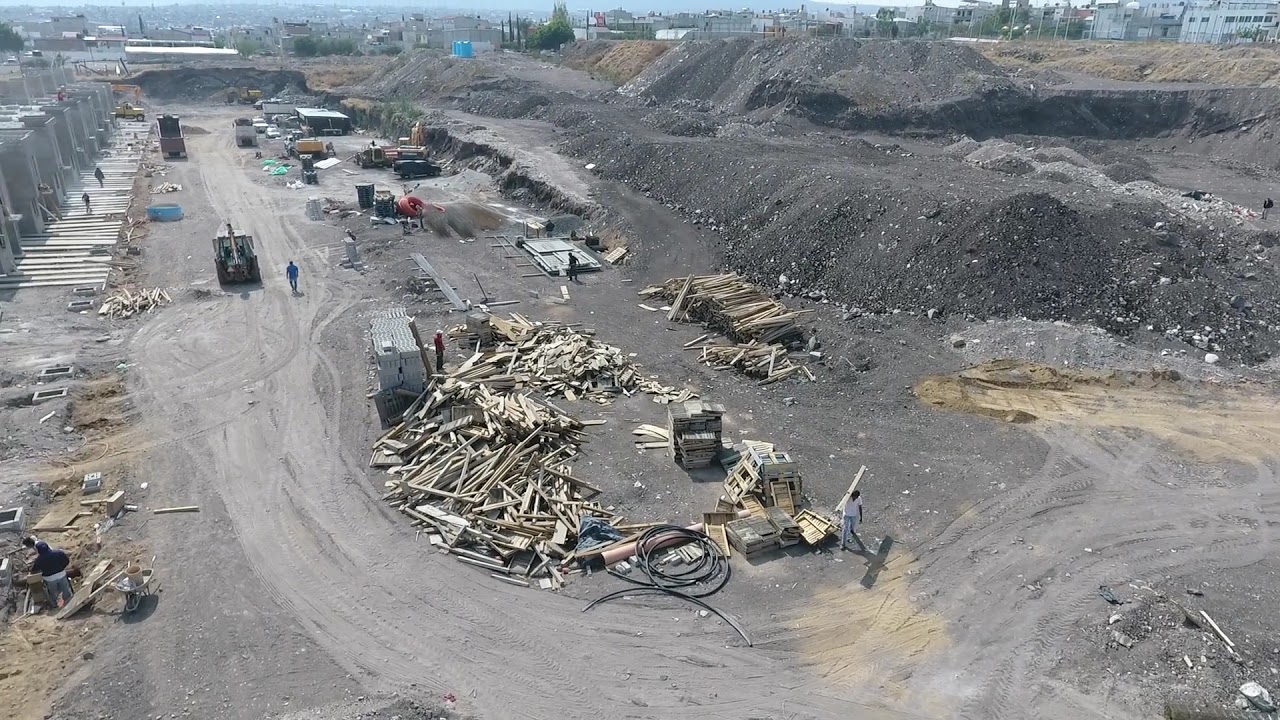The image depicts a large, busy construction site set within a deep excavation area, possibly for mining or building a substantial structure. The scene is coated with a palette of grayish-brown hues, featuring numerous piles of dirt, rubble, and rocks. Prominently visible are multiple stacks of lumber, crates, tubing, and wire scattered across the ground. In the background, large mounds of sand and dirt can be seen, with tall trees framing the horizon in blurred greens and grays.

Noteworthy activity includes several men working around the site. One man, wearing a blue shirt, strides from the rear to the front, while another, dressed in a white shirt and blue jeans, lifts a piece of wood from a nearby pile. Heavy construction equipment dominates the scene, including cranes, trucks, tractors, and garbage cans. Over on the left, wooden planks lie on the ground, and stone structures are visibly under construction. The site's industrial intensity is underscored by various materials like ropes and wires, indicative of the ongoing, rugged work. The time of day is clearly daytime, adding a bright and clear context to the bustling industrial environment.